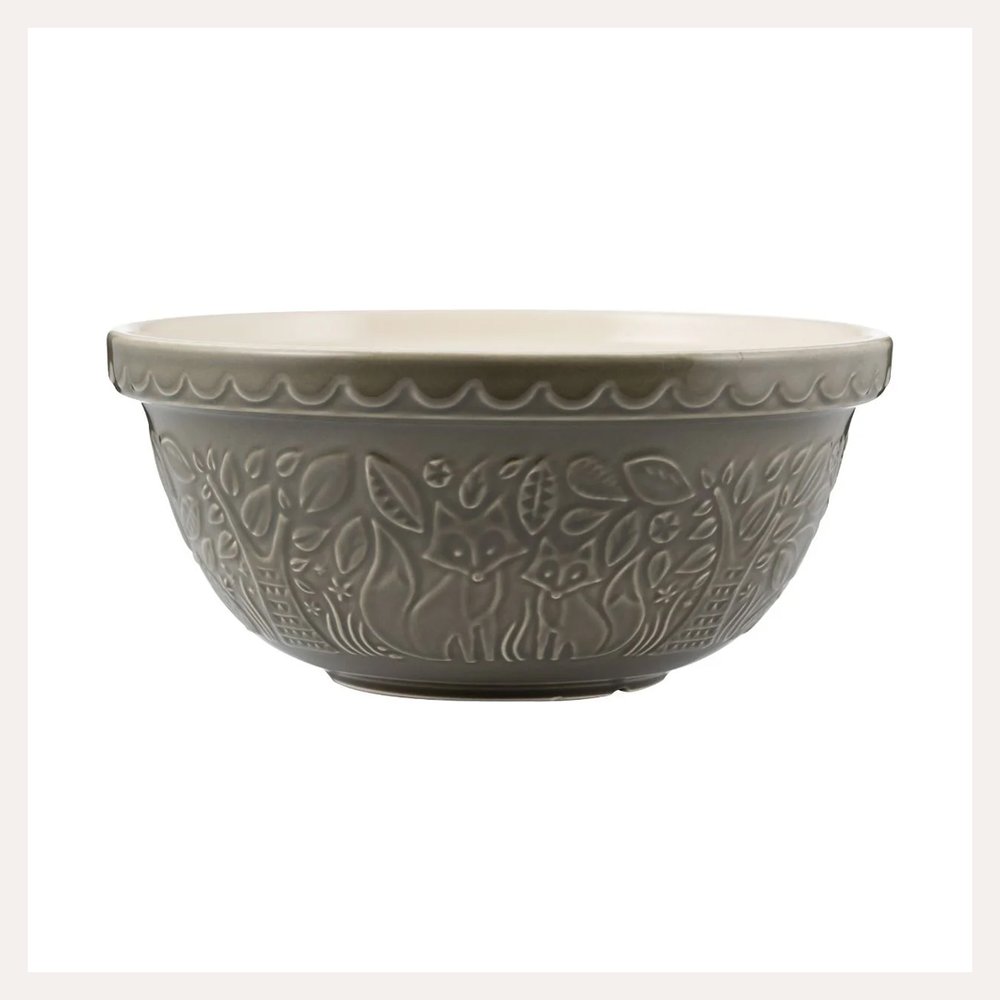This image depicts a dark gray ceramic mixing bowl with a decorative design. The bowl is centrally placed in a vertical, rectangular-shaped frame with a light gray border against a white background, making it appear as if it floats. The bowl features a flat, ruffled lid that matches its color and texture. Across the exterior, it showcases intricate carvings of a woodland scene: two stylized foxes situated at the bottom center, facing outward but with bodies turned towards each other. Surrounding the foxes are various leaves and tree trunks, providing a natural, forest-like ambiance. Additionally, the bowl's top rim is adorned with wave-like patterns, adding to its ornamental charm. The raised carvings are tactile, maintaining the same dark gray hue, contrasting subtly with the bowl's glossy glaze. Inside, the bowl appears white, enhancing the contrast with its dark exterior.